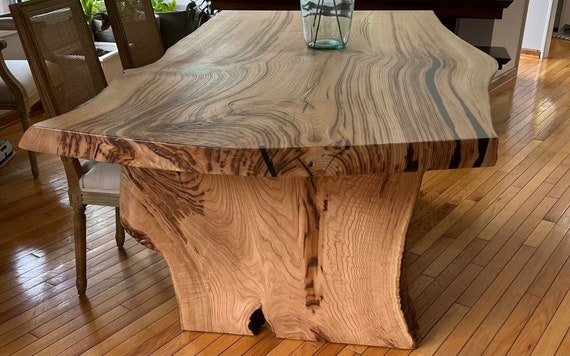This detailed image captures the rustic charm of a dining room centered around a striking wooden table made from a giant, natural slab of wood. Stretching from the bottom middle of the frame to the top, the table showcases a blend of dark grains with light brown and tan hues, emphasizing its handmade appeal. Supporting the sturdy tabletop is a single, solid piece of wood, similarly grainy and earthy-toned, that serves as the base. The floor beneath consists of narrow, light brown hardwood planks that complement the table's natural aesthetic. On the left side, two wooden chairs with fabric seats are neatly pushed in under the table. Atop the table rests a clear glass vase, partially visible and containing a few stems, adding a touch of elegance to this cozy indoor scene.